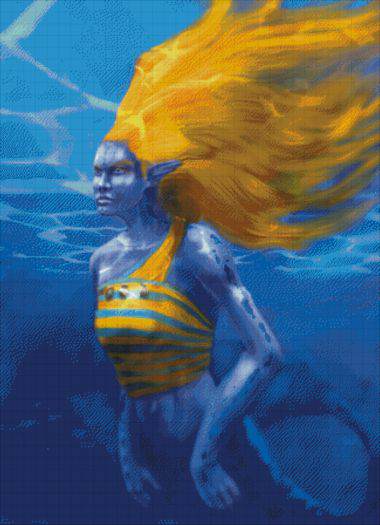This vertically oriented image, measuring approximately four inches tall and three inches wide, appears to be a painting or computer-generated artwork with a slightly pixelated texture resembling a blotchy canvas. It depicts an underwater scene, with a background that transitions from a deep dark blue at the bottom to a lighter blue at the top, enhanced by wavy gray lines that create the effect of being underwater. 

At the center of the image is a mermaid with blue skin and a serious, pointed face. She has long, pointed ears, reminiscent of an elf or fairy. Her bright yellow hair flows dramatically from the middle of the image to the upper right-hand corner. The mermaid is wearing a silver and yellow horizontally striped halter top, adorned with a single strap over her left shoulder that wraps around her back, revealing her midriff where her belly button should be visible. 

Her arms are spotted with silver patches, and a dark blue fishtail starts from the lower left-hand corner, blending seamlessly into the blue background, creating a blurred effect. The overall composition conveys a mystically serene underwater ambiance.